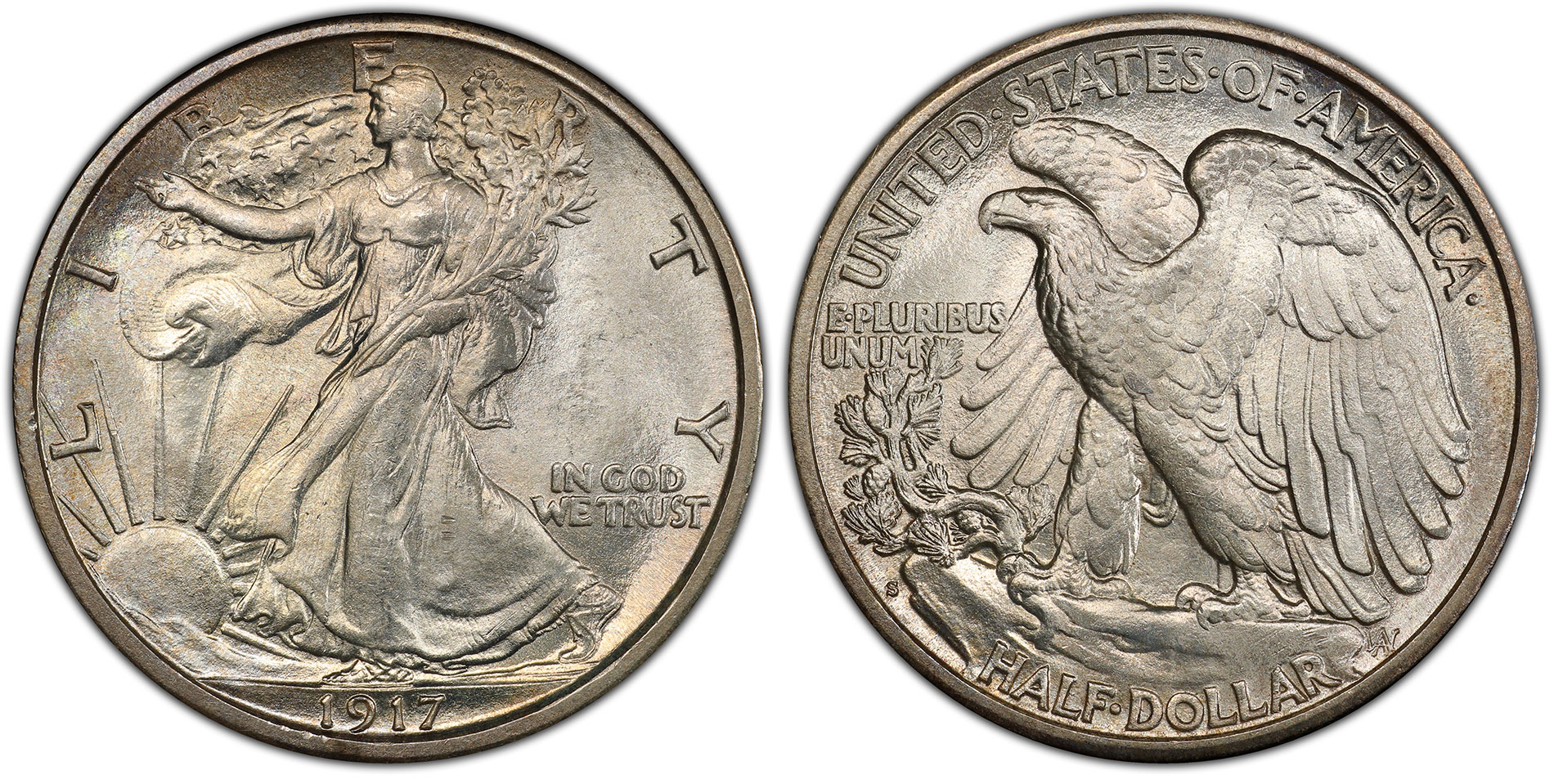This image showcases two pictures of a 1917 United States half-dollar coin, displaying both its obverse (heads) and reverse (tails) sides. On the left side of the image, the obverse side of the coin features a detailed depiction of Lady Liberty walking with an outstretched arm, draped in a flowing dress, and holding a bouquet of flowers. Above her head, "Liberty" is prominently inscribed, while the phrase "In God We Trust" is situated to her right, and the sun with radiating rays appears in the lower left corner. The year "1917" is stamped at the bottom of this side.

On the right side, the reverse of the coin displays an intricately engraved bald eagle perched on a rock, with a plant growing to its left. Surrounding the eagle are the inscriptions "United States of America" at the top and "E Pluribus Unum" beneath it, a Latin phrase meaning "Out of many, one." At the very bottom, the denomination "Half Dollar" is clearly marked. The entire coin is crafted in silver, showcasing fine details in its engravings.